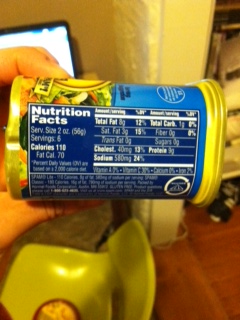This photo captures a close-up view of a container's side, specifically focusing on the nutrition facts label. The background features a brown wooden floor and an ivory-colored wall. Some undefined gold-colored object is visible at the bottom of the image. A human hand, fair-skinned and belonging to a person who is left-handed, is holding the container. The hand is positioned to tilt the container sideways, making the nutrition facts readable. 

Despite the top of the container being out of frame and the focus being somewhat blurry, some text on the label is discernible. The nutrition facts indicate a serving size of two ounces, with approximately six servings per container. Each serving provides 110 calories, with 70 of those calories coming from fat. Additional nutritional information includes:

- Total Fat: 8 grams
- Total Carbohydrates: 1 gram
- Cholesterol: 40 milligrams (estimated)
- Protein: 3 grams
- Sodium: 580 milligrams

The nutrition facts section stands out with its dark blue background and white lettering, while the container's lid is a noticeable yellow.